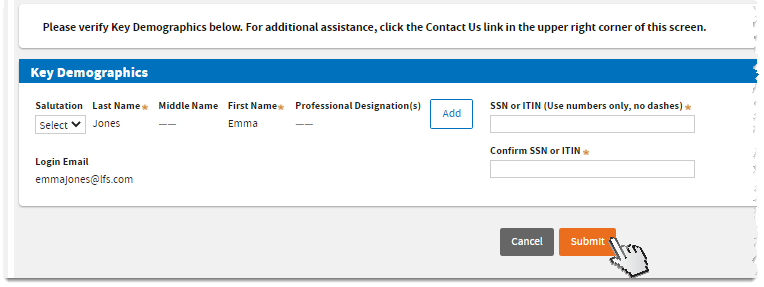In the image, the top section features a white box with the message "Please verify key demographics below." For additional help, there is a "Contact Us" link located in the upper right corner of the screen. The header has a dark blue border with the text "Key Demographics" in white. Below this, "Salutation" appears with a corresponding drop-down menu labeled "Select."

To the right, "Last Name" is marked with an asterisk, followed by the text "Jones." Underneath, "Middle Name" is displayed with two dashes below it, indicating no information provided, and "First Name" accompanied by an asterisk displays "Emma." The "Professional Designation" field also has two dashes to indicate no data entered. 

A white box with a blue border containing the label "Add" is visible, and to the right, the field for "SSN or ITIN" is indicated, with instructions to use numbers only, without dashes. This is marked with an orange asterisk, denoting it as a mandatory field, along with a text box below it for input. Additionally, another instruction reads "Confirm SSN or ITIN," marked with an orange asterisk and a text box for confirmation below it.